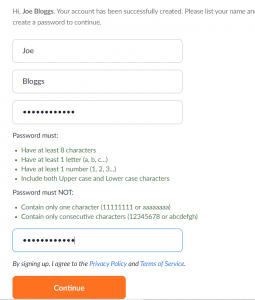The image depicts a slightly blurred sign-on screen with a welcome message addressed to Joe Blogs, indicating that his account has been successfully created. The screen prompts the user to enter their first and last name, which Joe has already done, listing "Joe" in the top input field and "Blogs" in the field below. There's a hidden password field with an indicator showing that Joe has entered a password. Instructions beside the password field specify that the password must be at least eight characters long, contain at least one uppercase and one lowercase letter, and include at least one numeral—for example, A, b, and 1. The guidelines also note that passwords cannot contain repetitive characters. An orange button labeled "Continue" is visible, inviting the user to proceed with the account setup process.